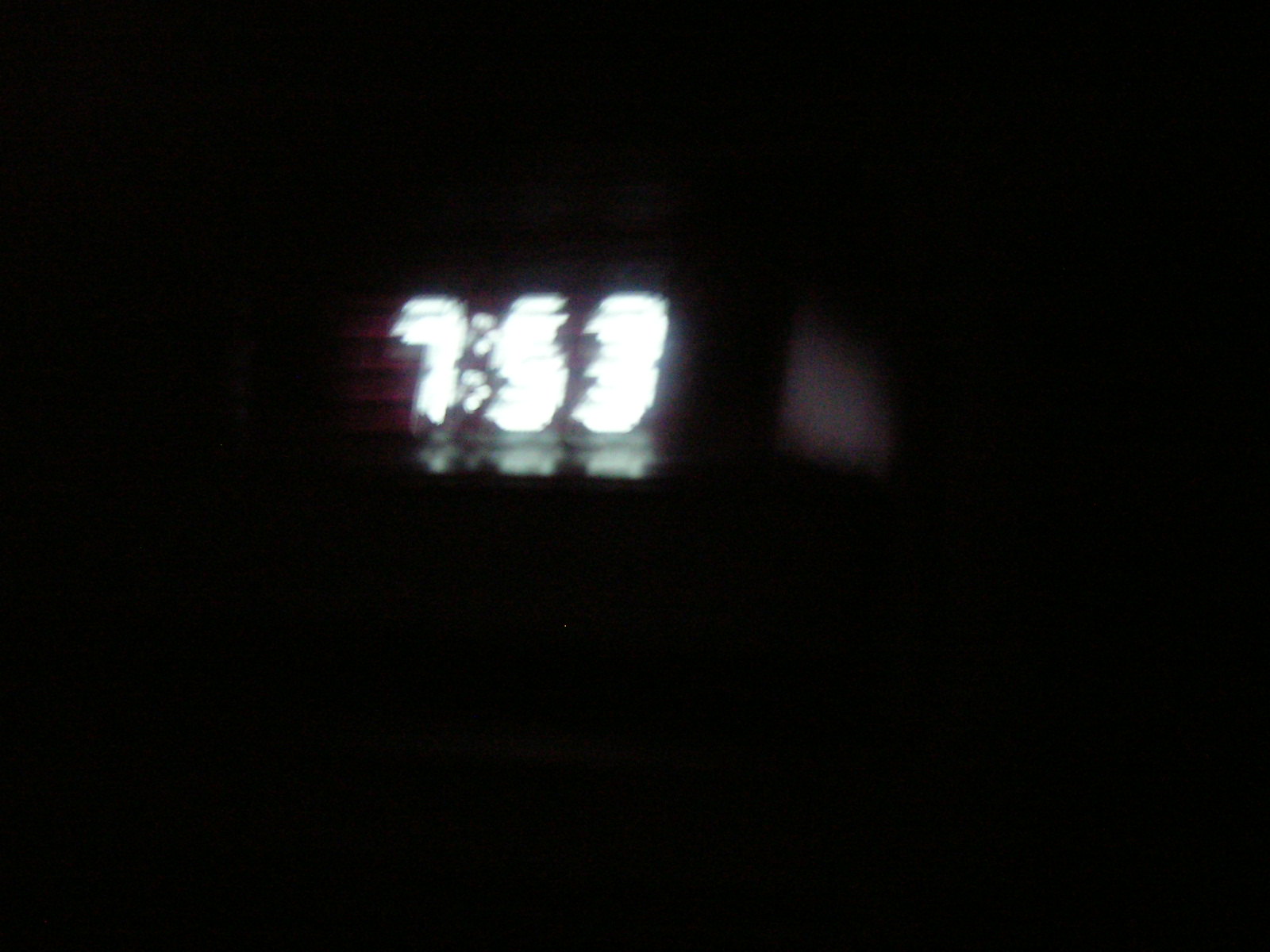Blurry photograph showing a digital clock with a rectangular body set against a pitch-black background. The clock, which appears to have a black face and white numbers, displays the time as "7:53." The image is distorted, possibly due to camera shake, creating a heavy blur around the numerals and making them difficult to discern. There is some reflection and a hint of white color on the clock's body, adding to the indistinct, ethereal quality of the photograph.